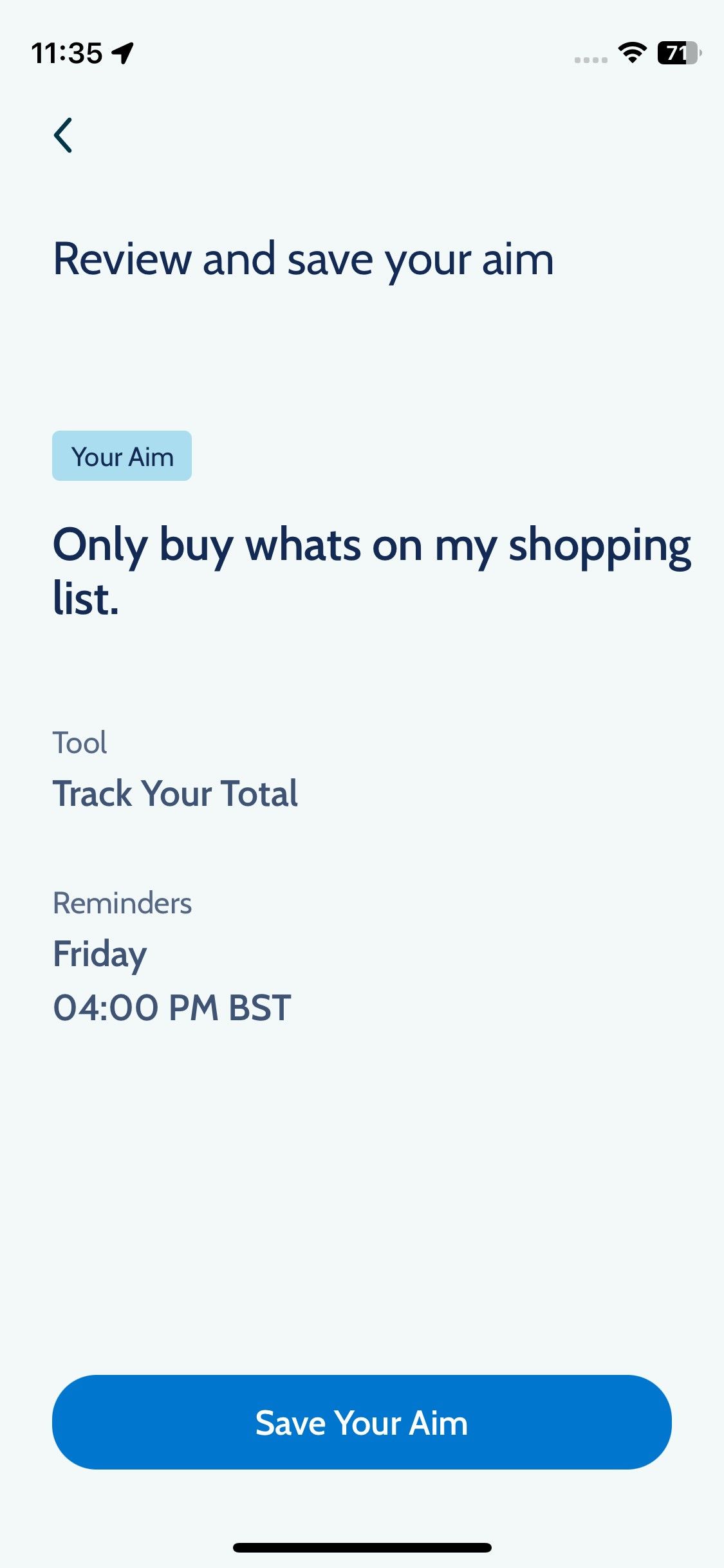The cell phone screenshot features several elements organized in a clean, structured manner:

- **Upper Section:**
  - On the upper right-hand side, common cell phone icons are visible.
  - On the upper left-hand side, the time is displayed.

- **Navigation and Heading:**
  - Below the time, a black back arrow is visible, followed by a space.
  - Left-justified, the text "Review and Save Your Aim" is written in black font.

- **Buttons and Headings:**
  - Four spaces below, there is a small aqua-blue button with black font that reads "Your Aim."
  - A space beneath the button, a larger black font heading states: "Only Buy What's On My Shopping List."

- **Sections and Subheadings:**
  - After two spaces, there is a smaller, lighter font that labels the section as "Tool."
  - Below this, a thicker, bolder, and slightly larger font reads: "Track Your Total."

- **Reminders:**
  - Followed by two spaces, the section labeled "Reminders" appears.
  - Below "Reminders," the day "Friday" is indicated.
  - Subsequently, the time "4 p.m. BST" is mentioned.

This detailed caption covers all aspects of the visual elements present in the cell phone screenshot.